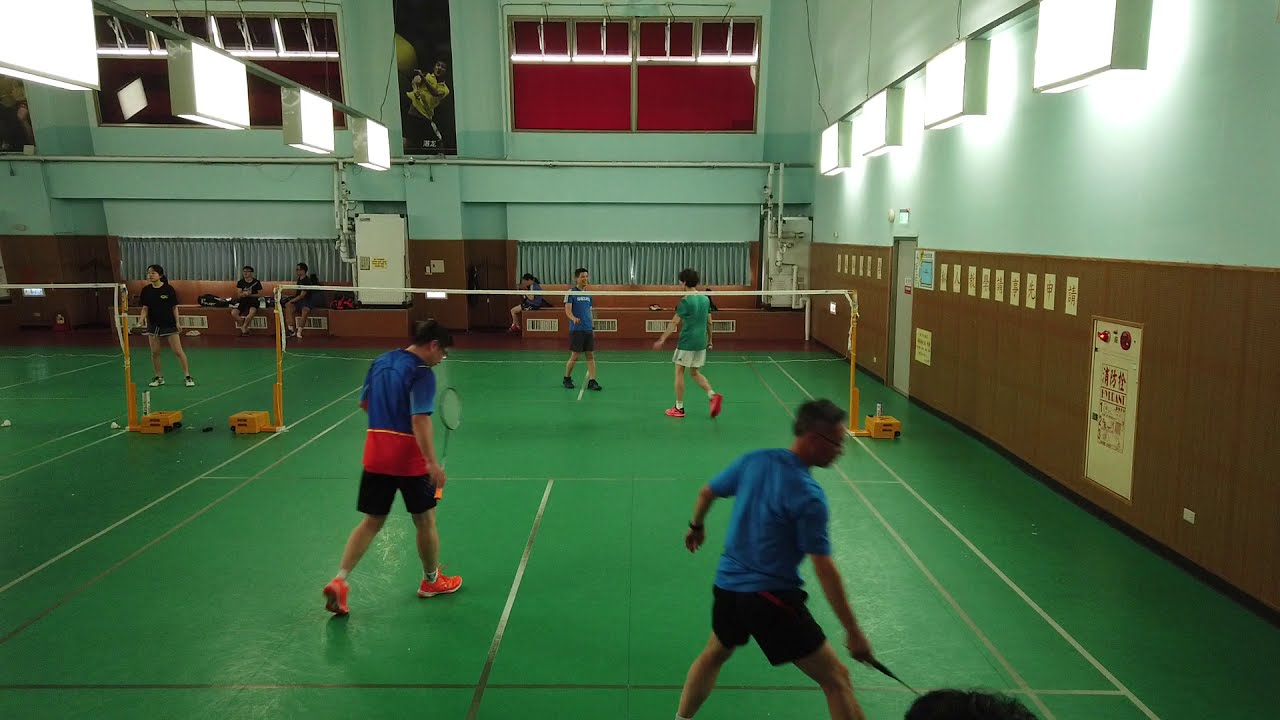In this indoor recreational center, we observe a lively game of badminton played on a green court marked with silver boundary lines. The setup includes multiple badminton courts, with the focus primarily on one against the wall, and a partial view of another adjacent court. The walls are primarily white, accented with wood grain decorations on the right side. Additionally, white posters bearing Asian characters indicate an Asian country setting, and the windows are covered with red curtains.

On the featured court, four men are engaged in a paused game. Closest and to the right, one man, wearing a blue shirt, orange and black shorts, and orange shoes, holds a racket in his right hand. His partner, slightly ahead, is dressed in a blue shirt and black shorts, with a watch visible on his wrist. Across the net, one opponent wears a green shirt and white shorts with orange shoes, while his teammate sports a blue shirt, black shorts, and black shoes. The net has yellow railing and a white mesh.

Surrounding the players, additional details include blacked-out windows with red curtains, and posters of players adorning the walls beneath a series of large rectangular ceiling lights. The high ceilings and potential wooden seating in the background add to the spacious and dynamic atmosphere of the scene.